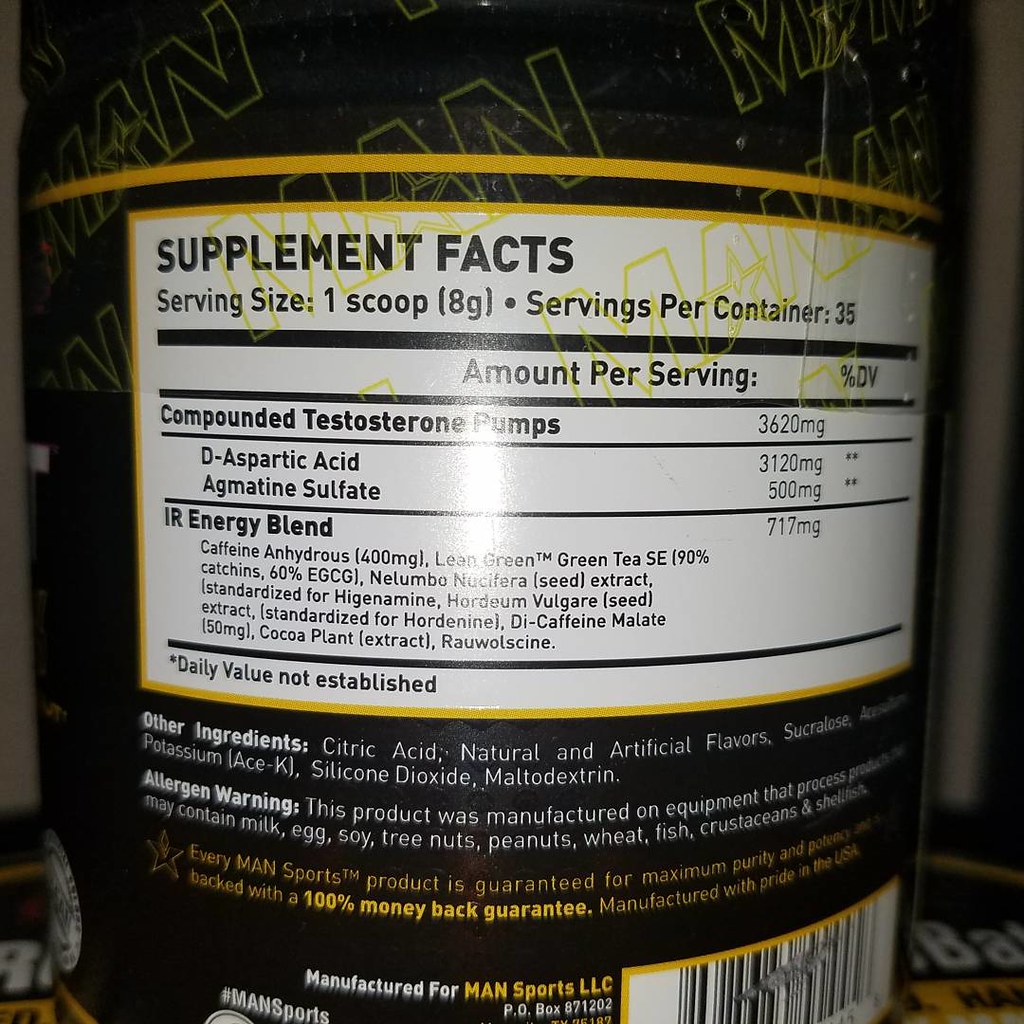The image features the back of a black cylindrical container. The top of the label prominently displays the outline of the word "MAN" in large yellow lettering, followed by a yellow bar beneath it. Below the bar, the "Supplement Facts" label is clearly visible, indicating a serving size of 1 scoop (8 grams) and a total of 35 servings per container. The label goes into detail about the ingredients, listing components like "compounded testosterone pumps" and "IR energy blend."

Outside the main supplement facts box, in white lettering, are other ingredients and allergen warnings. A star icon highlights that every MAN SPORTS product guarantees maximum purity and potency, supported by a 100% money-back guarantee despite some illegible text. At the bottom of the label, it states that the product is manufactured for MAN SPORTS LLC, and a barcode is also present in the lower section.